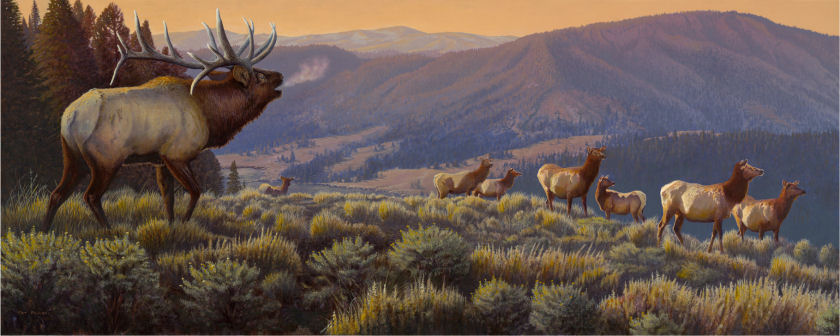This is a highly detailed and realistic painting depicting a serene, sun-kissed landscape featuring a majestic herd of elk. The primary focus is a large male elk with prominently curved antlers, standing on the left side of the image. This stag, half brown and half white with brown legs, is exhaling visible breath into the cool air. To the right, slightly in the background, a group of seven smaller elk, likely females or juveniles, share the same brown and white coloring. They are scattered across a lush, green pasture-like hillside adorned with various shrubs. The background reveals a beautiful, expansive mountain range with scattered trees, suggesting a dense forest. The sky above is a warm shade of orange, indicating a sunset, which casts a golden glow across the scene and the mountainous horizon in the distance.